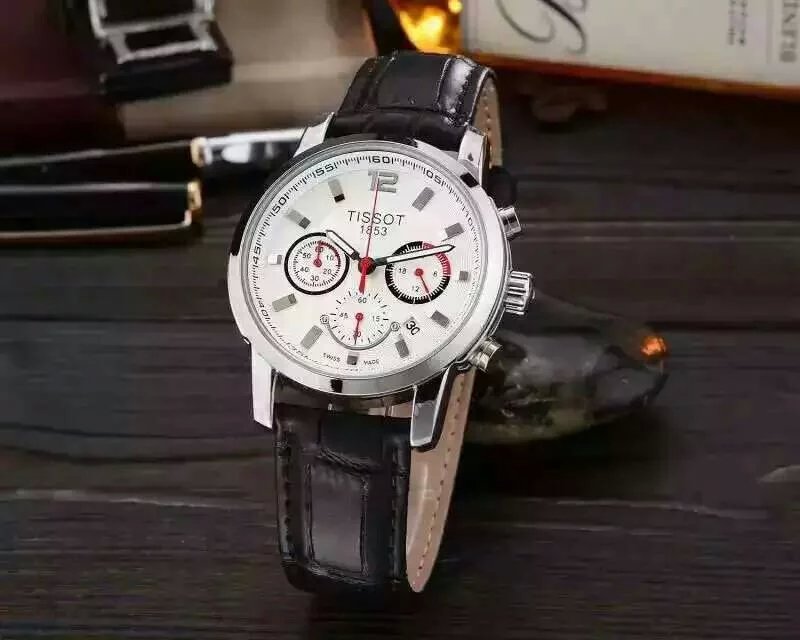This detailed photograph showcases a sophisticated wristwatch artfully positioned on a rich, dark wooden table. The watch features an elegant black leather band with a contrasting tan interior, lending a touch of classical refinement. Its pristine white face is encased in a sleek silver frame, accentuated by a polished silver bezel. The watch face is meticulously designed with gray numerals, prominently displaying the number 12, while understated gray lines denote the remaining hours. Three smaller sub-dials add complexity and functionality to the design. In the backdrop, a product label strikes a classic note with black cursive writing on a white surface set against a shimmering gold background. Additionally, a square object in black and silver occupies the upper left corner, contributing to the composition. A pair of stylish black and gold sunglasses rests casually behind the wristwatch, completing the scene with an air of effortless elegance.